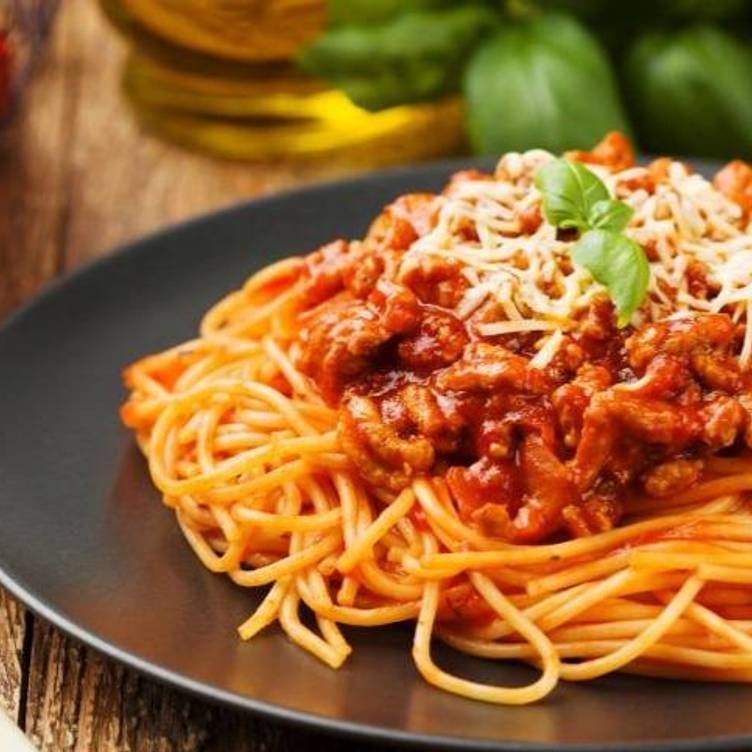This photograph is a close-up shot of a dish of spaghetti Bolognese presented on a rustic wooden surface, possibly a table or countertop. The setting hints at either a kitchen or a restaurant. The image prominently features a round, black plate positioned towards the bottom right of the frame, with the spaghetti extending slightly off to the right. The spaghetti is generously coated in a rich, red tomato-based sauce and is topped with a hearty dollop of Bolognese sauce made from ground beef. Grated Parmesan cheese is sprinkled over the top, and a fresh basil leaf adds a touch of elegance to the dish. In the blurred background, to the upper right of the image, additional basil leaves and a partially visible jar, likely containing olive oil, can be seen. The overall color palette includes various shades of brown, black, red, green, yellow, and orange.